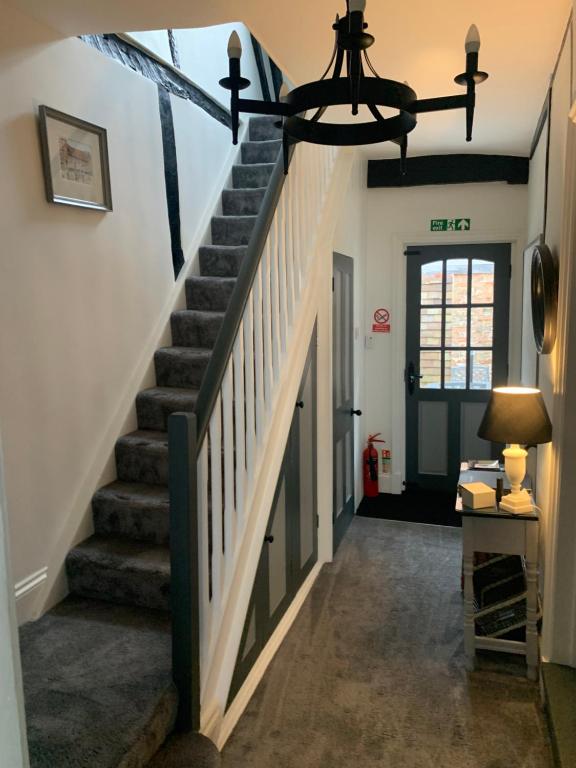The image depicts a narrow stairway on the left side, leading up to the next floor, covered in grayish carpet. The main focus is the hallway of a house, predominantly white in color, with pristine wooden floors. Toward the right center of the hallway stands a back door, adorned with glass paneling, allowing natural light to filter in. A light fixture on the ceiling illuminates the space, and a neatly placed desk adds a functional touch to the hallway scene.